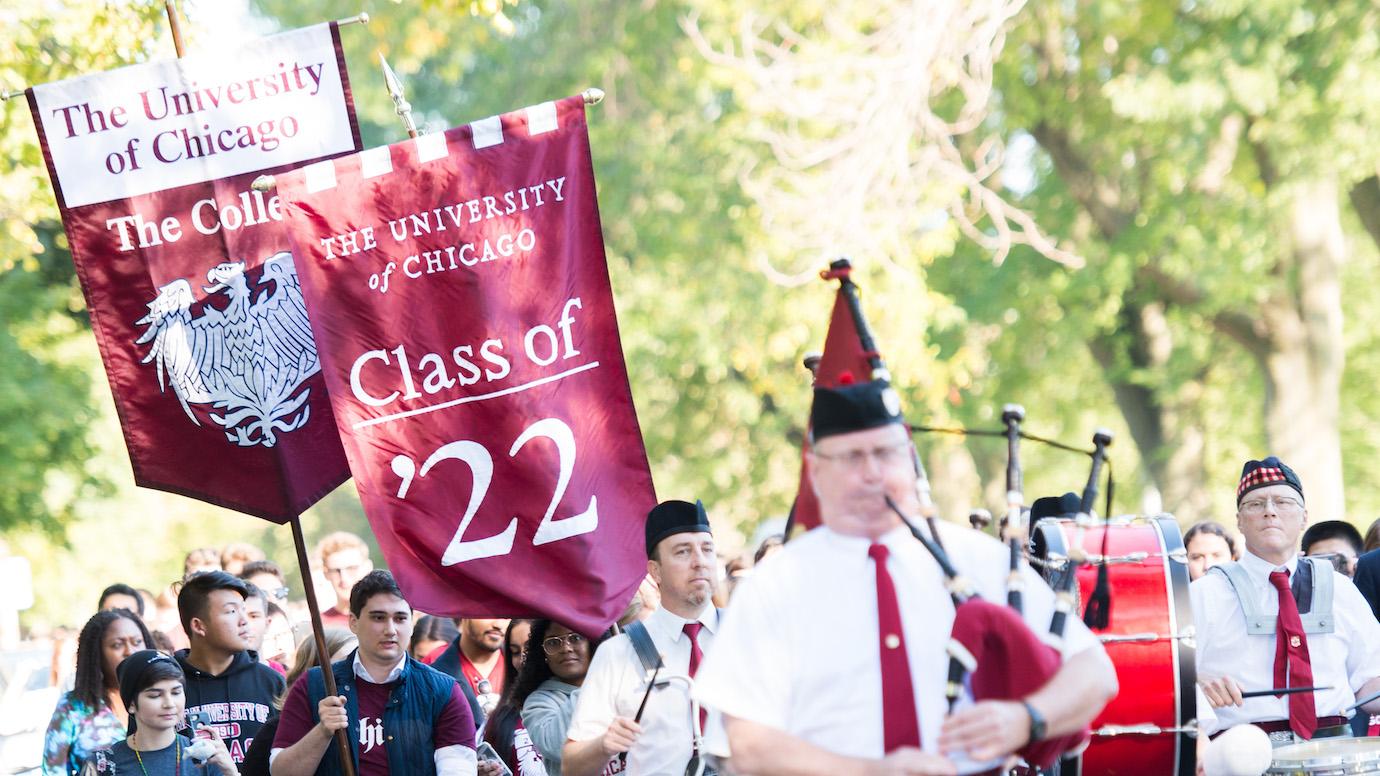This photograph captures a vibrant parade at the University of Chicago. Dominating the foreground is a man energetically playing red bagpipes, with his cheeks puffed out and eyes scrunched in concentration as he blows into the instrument. He wears a red tie, black hat, and glasses, adding distinct elements to his traditional appearance. Behind him, there are several drummers clad in coordinated attire featuring red ties, white shirts, and flat black hats. Their drums vary, including snare drums and a notable large red and black bass drum.

Following the musicians is a diverse group of students, representing various ages and ethnicities, dressed casually in hoodies and beanies. Several of these students carry prominent red banners on large wooden sticks. One banner announces "University of Chicago, Class of 22," while another declares "University of Chicago, The College," featuring an emblem of an eagle in white. The backdrop of the scene is filled with green, leafy trees that are slightly out of focus, emphasizing the lively and communal atmosphere of the parade.